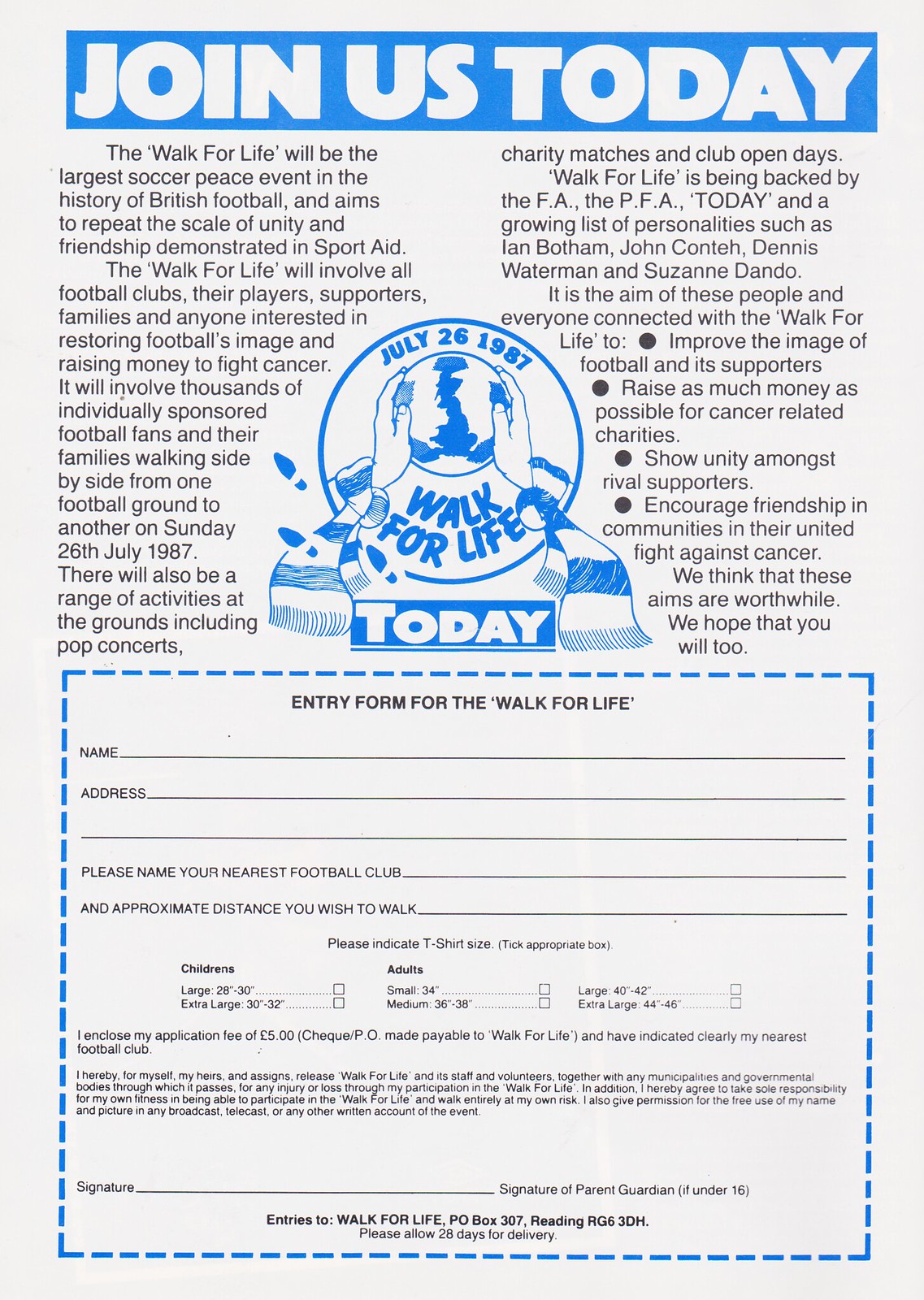This vintage advertisement, likely clipped from a magazine due to its blue and white print on a white background, promotes the "Walk for Life" event that took place on July 26, 1987. The ad's top heading, displayed in large, white, bold letters on a light blue background, invites readers to "Join Us Today." Below the heading, two columns of text describe the event's details. The Walk for Life is poised to be the largest soccer peace event in the history of British football, aiming to emulate the unity and friendship demonstrated in Sport Aid. The walk involves all football clubs, their players, supporters, families, and anyone dedicated to restoring football's image and raising funds to fight cancer. Participants, including thousands of individually sponsored football fans and their families, will walk from one football ground to another. The event promises various activities at these grounds, such as pop concerts, charity matches, and club open days.

Centrally placed between the two text columns is a round emblem featuring two hands holding a globe, with the date "July 26, 1987" above and "Walk for Life" below. Below this emblem, the word "Today" is prominently displayed. The ad mentions the event's backers, including the FAA, PFA, Today, and notable personalities like Ian Waltham, John Kattay, Dennis Waterman, and Suzanne Dardo. The goals of the Walk for Life include improving football's image, raising money for cancer-related charities, fostering community unity, and encouraging friendship. 

At the bottom of the ad, there is an entry form with dotted blue lines intended for readers to fill out with their personal information if they wish to participate in the charity walk. This detailed solicitation underscores the collective effort to unify football supporters and fight cancer through this historic event.